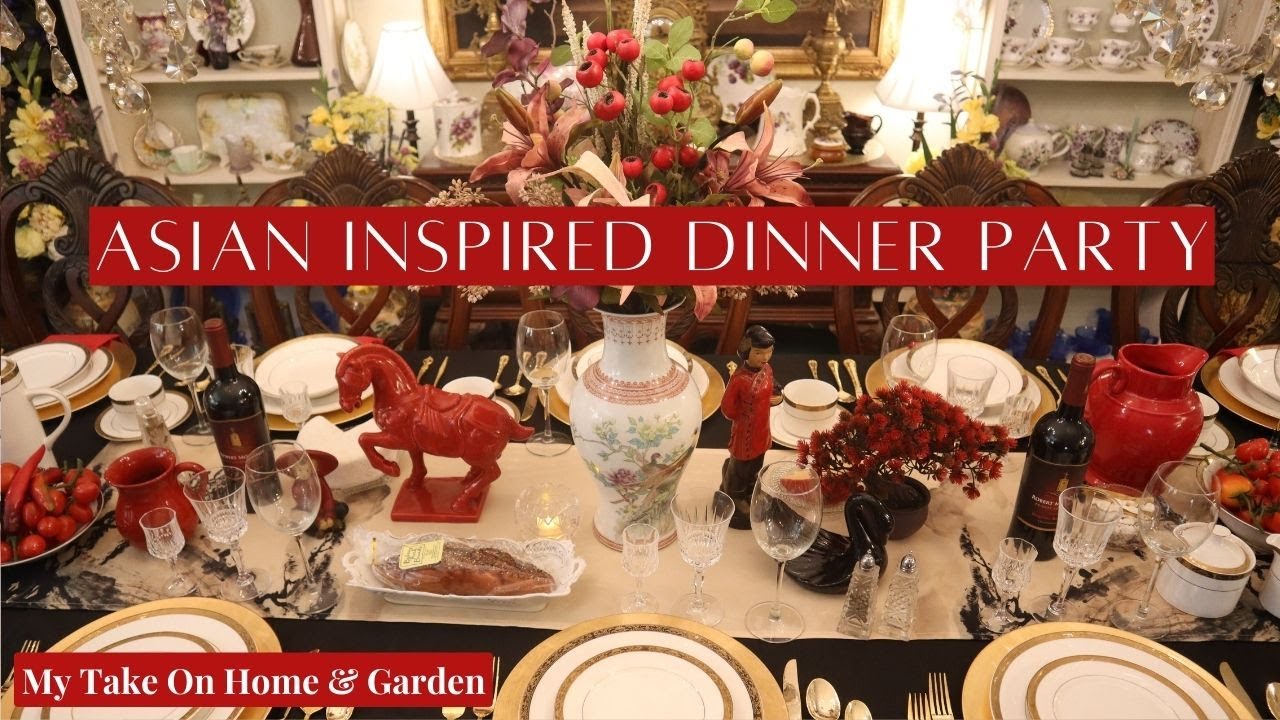The image appears to be a professionally taken photograph, possibly an advertisement, featuring a lavishly decorated table set for an "Asian-inspired dinner party." At the top center, there is a red banner with white text reading "Asian-inspired dinner party," while the bottom left corner features another red banner with white text saying "my take on home and garden." The tablescape is ornate, boasting a striking and colorful centerpiece—a white vase with floral designs that include green, red, and yellow hues, filled with an array of leaves, flowers, and small red bulbs. Flanking the table are decorative elements such as black vases with red accents, a solid red statue of a horse, an Asian statue, a bowl of red peppers, and a large red pitcher next to bottles of wine. On the table, a black tablecloth is overlaid with a white runner, complemented by white China dishes and assorted glassware. The vibrant red and white palette is prominent throughout, accented by a small black statue resembling a duck. The meticulous arrangement and rich details make the scene reminiscent of a magazine spread.